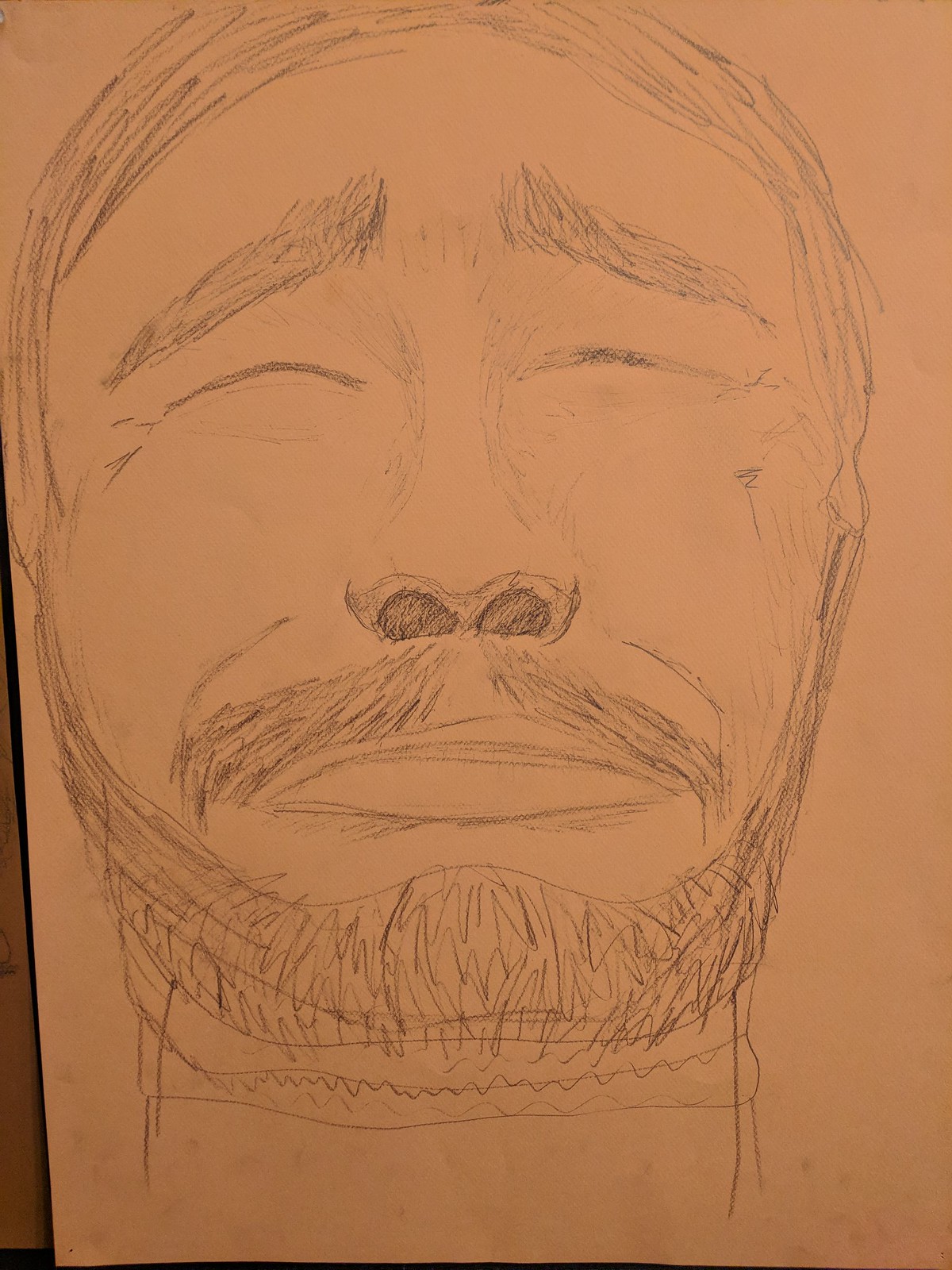This is a digital photo of a hand-drawn pencil sketch. The drawing depicts a man in apparent pain or emotional distress, as suggested by his closed eyes, flared nostrils, and high, arched eyebrows. His facial expression indicates an intense, possibly sorrowful state. The man is characterized by his short hair, bushy eyebrows with a thin unibrow, a substantial nose with heavily shaded-in nostrils, thin mustache that sparsely covers the center above his lips, and a full beard. The detailed contours of his face, including his high cheeks, reinforce the sense of his discomfort. The sketch is rendered on what appears to be cream or whitish cardstock. The background of the digital photo, seen in the lower left, includes a darker tan-colored wall. This intricately drawn image is a monochromatic composition, emphasizing the stark, raw emotion through meticulous pencil shading and texture.